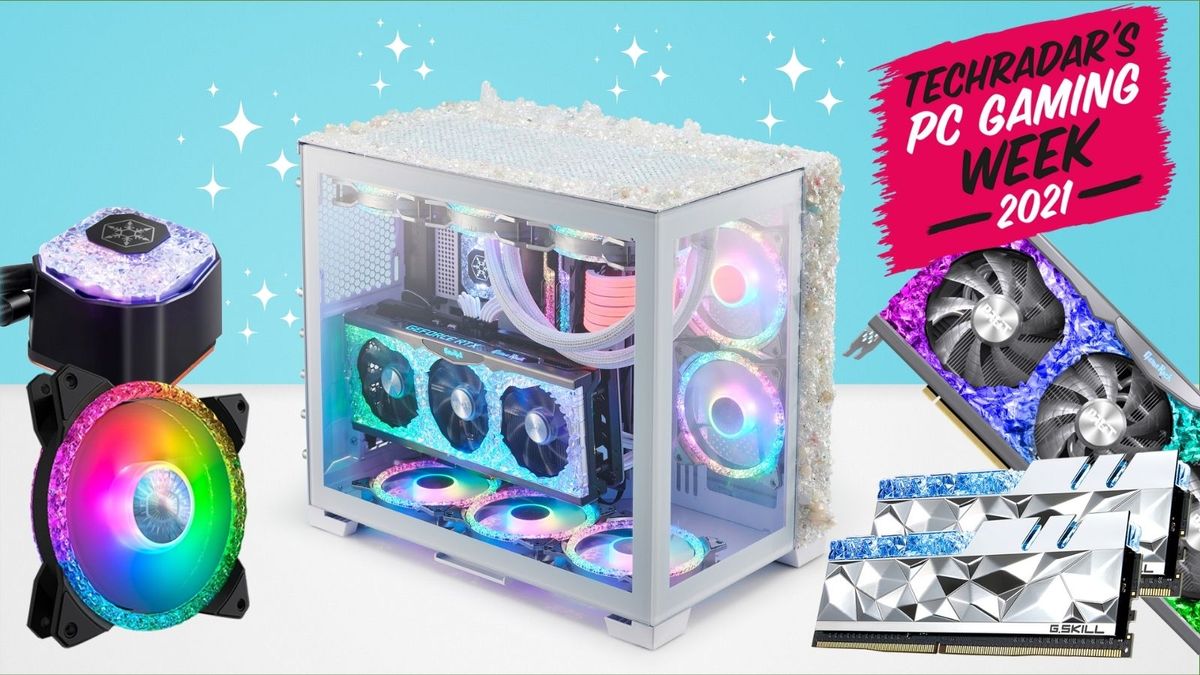The image features a top half with a light turquoise background adorned with sparkling white stars shaped like tiny diamonds, transitioning into a plain white bottom half. Central to the image is a see-through rectangular box, housing vibrant rainbow-colored discs. To the left of this clear box is a black gadget with a shiny purple top, displaying another upright rainbow disc. The right side showcases a dark pink square inscribed with "Tech Raiders PC Gaming Week 2021". Beneath this, a colorful square contains black circular patterns. Overall, the scene combines elements of PC components and vibrant colors against a fantastical backdrop.